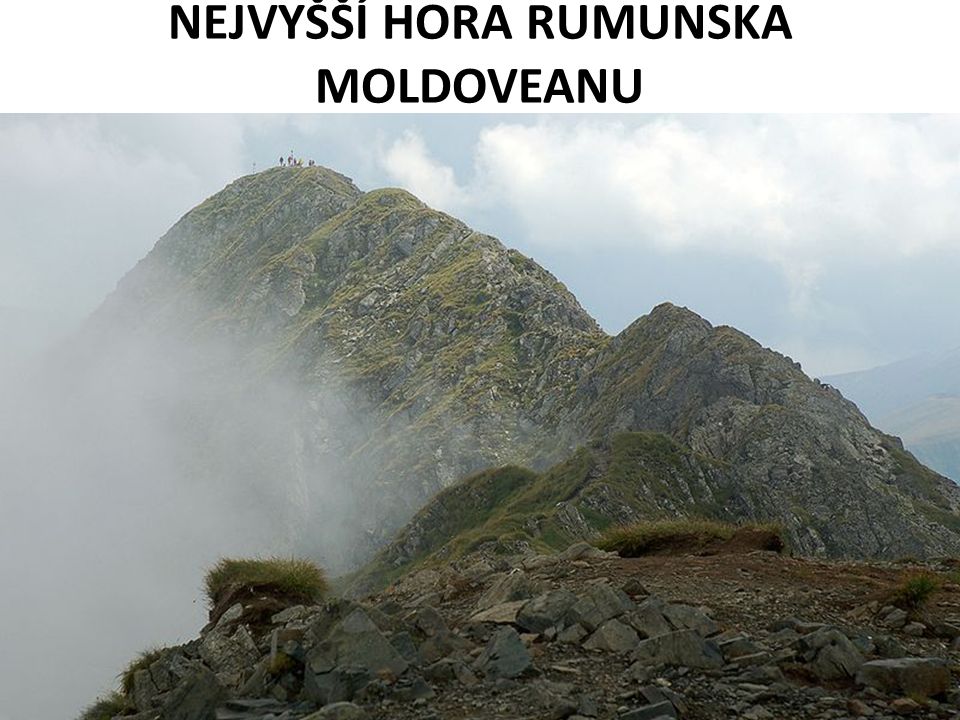The image depicts a rugged and steep mountainous region labeled at the top in a non-English language, ending with "Neve Jisi Hora Rumunska Moldovano." The foreground showcases a prominent mountain peak characterized by rough, barren rocky surfaces interspersed with sparse grass and moss. The imposing cliffs and crags give the impression of a challenging and potentially dangerous climb, devoid of any established hiking trails. In the background, three additional large mountain peaks stretch across the horizon. The tallest peak, farthest from the camera, subtly reveals a small gathering of people at its summit, though the distance makes it hard to discern their exact number. The overall atmosphere is shrouded in fog and clouds, suggesting a high altitude with dense, misty air. To the left of the image, the mountain range fades into white smoke, while to the right, the light blue sky peeks through the cloud cover, creating a striking contrast amidst the peaks.